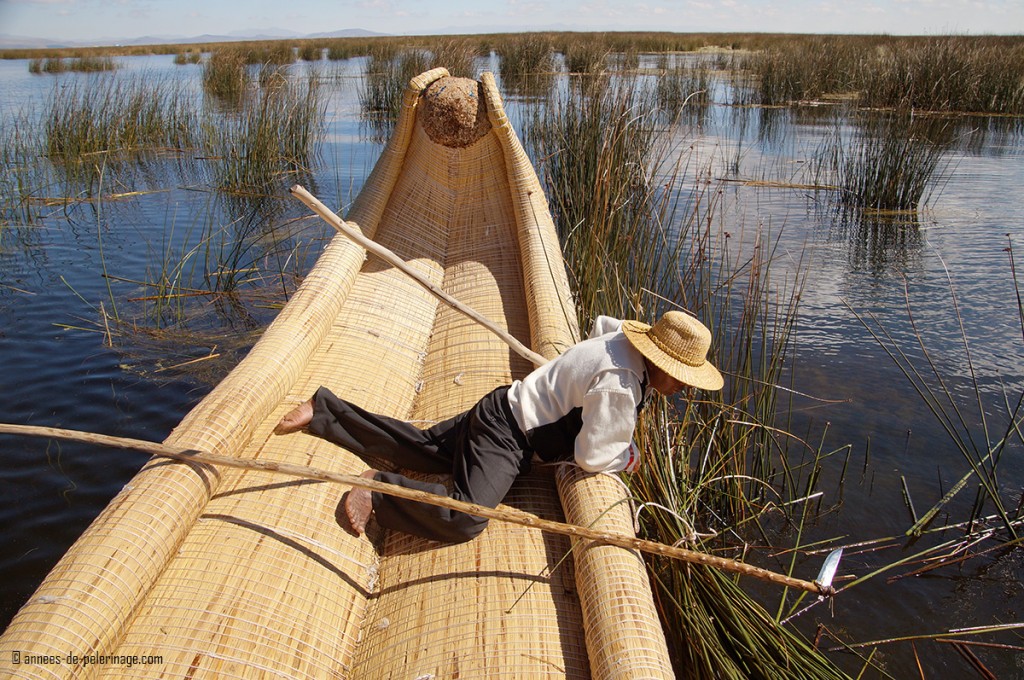This horizontal rectangular photograph depicts a man in a large, shallow wooden boat, resembling an oversized canoe. The boat, adorned with a brown ball-like stone at the curved top, appears to be constructed from light, golden tan plant material. It is nestled among tall green reeds in a calm river with gentle ripples. The man, dressed in black pants, a white pullover jacket, and a large, round wicker hat styled like a sombrero, is lying on his stomach across the boat's curved surface. He peers intently into the water, propped up on his elbows. On either side of him rest two long poles, one equipped with a silver blade, suggesting he might be spearfishing or harvesting aquatic plants. Text at the bottom reads, "and he's to pedagogy calm," hinting at his focused, methodical activity. The lush, watery landscape evokes a scene reminiscent of the Everglades, yet with an Asian ambiance.